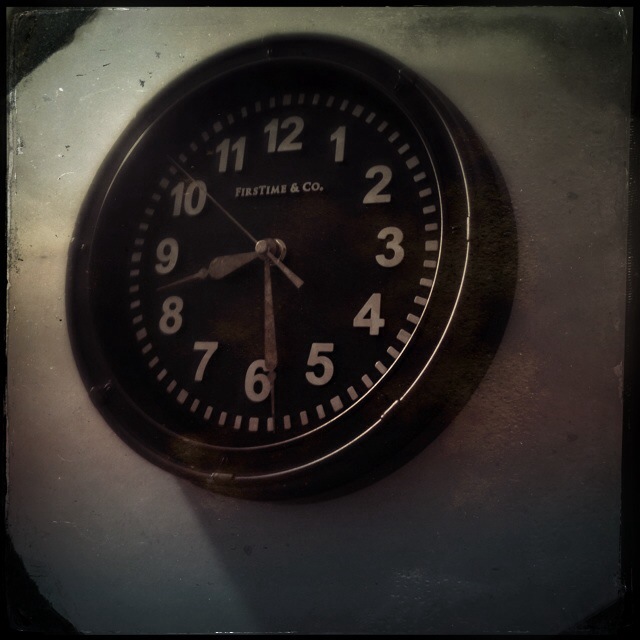A sleek, modern wall-mounted clock stands out against a light gray wall, which features distinctive shadowing in each of its four corners, casting a dramatic black hue. The clock itself is round with a shiny black frame that adds a touch of sophistication. Its face is entirely black, adorned with stark white numbers for clear readability. Surrounding the numbers, small white dots mark each passing second. The clock's minute and hour hands are a robust dark gray, providing a bold contrast against the black background. An elegant, needle-like second hand, also in dark gray, sweeps around the face with precision. Beneath the number 12, white text reveals the manufacturer's name. The time depicted on the clock is 8:29.